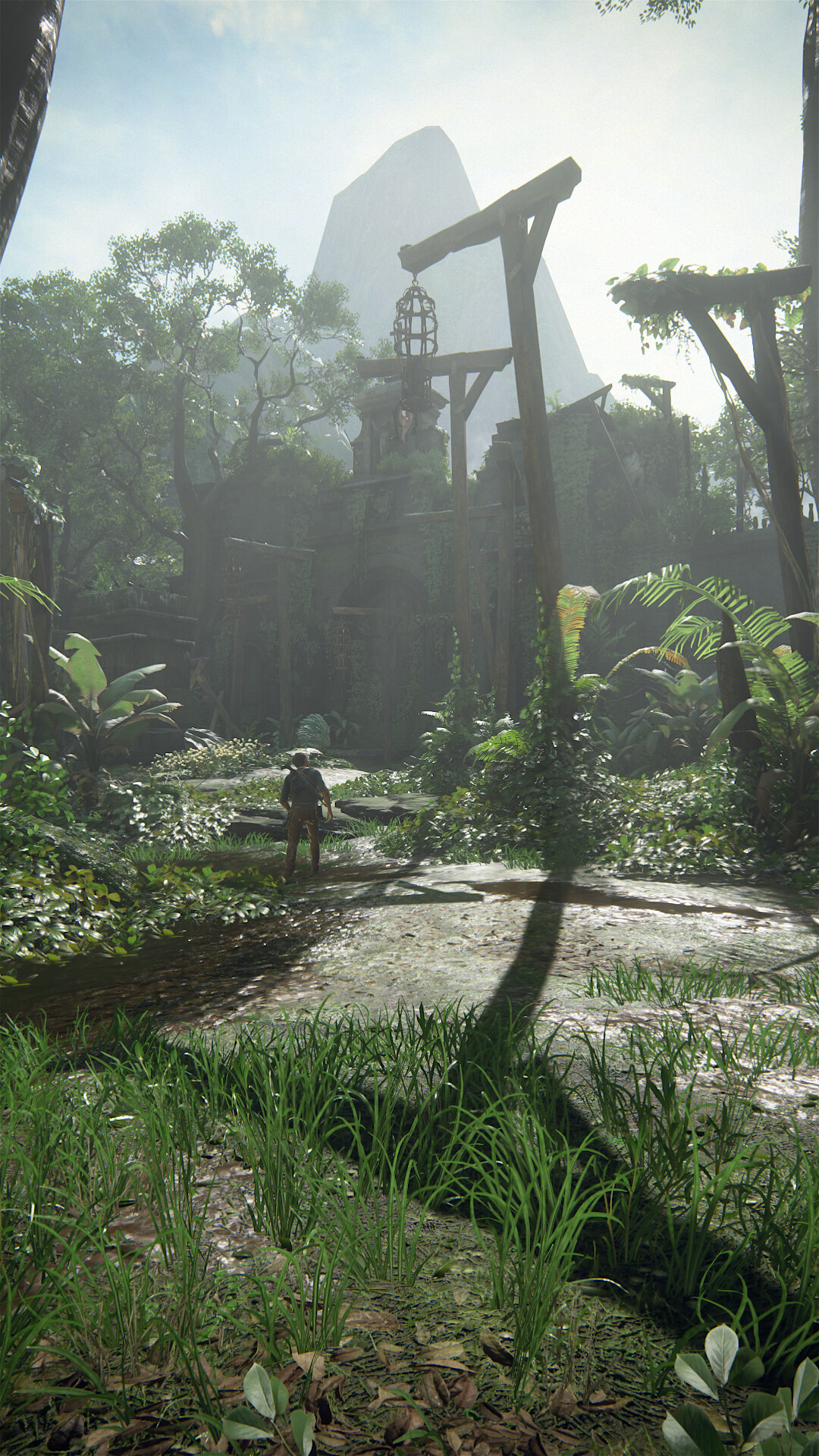The image captures a serene forest scene viewed from above, emphasizing an open clearing within the dense foliage. In the background stands an imposing building whose entrance is framed by long, stone walls that rise majestically from the bottom of the image to converge at the center where the building is located. This architectural feature creates a grand, almost ceremonial, pathway leading to the entrance. Along this pathway, a series of large wooden poles are strategically placed on both sides. These poles are adorned with structures resembling birdcages, which appear to be lantern holders. At the heart of the scene, in the distant center of the pathway, a solitary figure is visible, rendered almost minuscule by the scale of their surroundings, adding a sense of depth and perspective to the tranquil tableau.